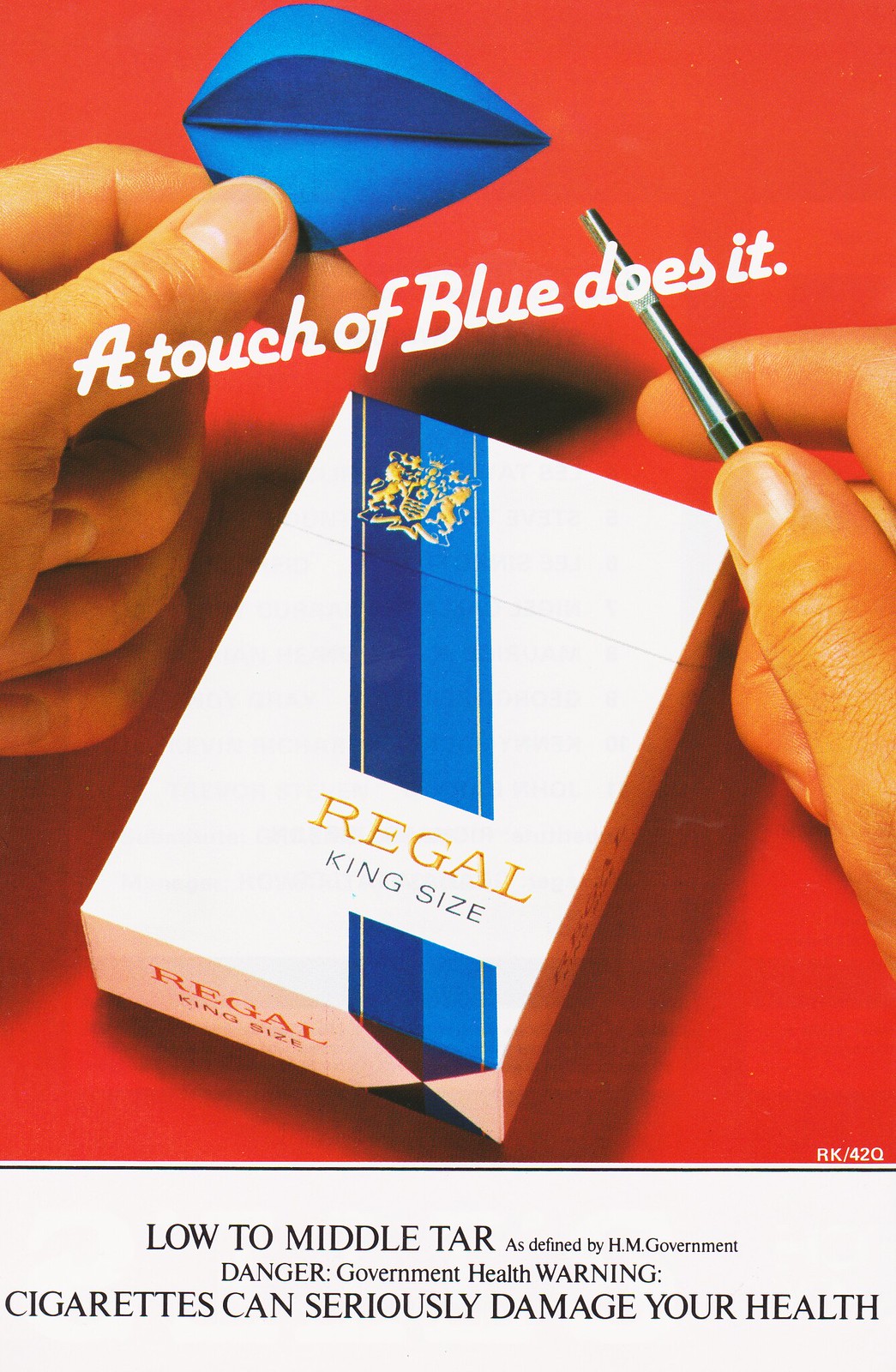The advertisement is a color image with a bold red background, centrally featuring a white box of Regal king-size cigarettes adorned with both dark blue and light blue diagonal stripes, and hints of gold. The focal point also includes two hands; the left hand is holding what appears to be a blue, folded piece of paper resembling a dart feather, while the right hand holds a black pointed object, likely the dart head. The text prominently displayed above the cigarette package reads, "A touch of blue does it." Below the image, additional text highlights the product as "low to middle tar" with an explicit government health warning: "Danger, Government health warning. Cigarettes can seriously damage your health." The advertisement is styled as a magazine print, with all elements harmoniously emphasizing the cigarettes amid the vivid red background.